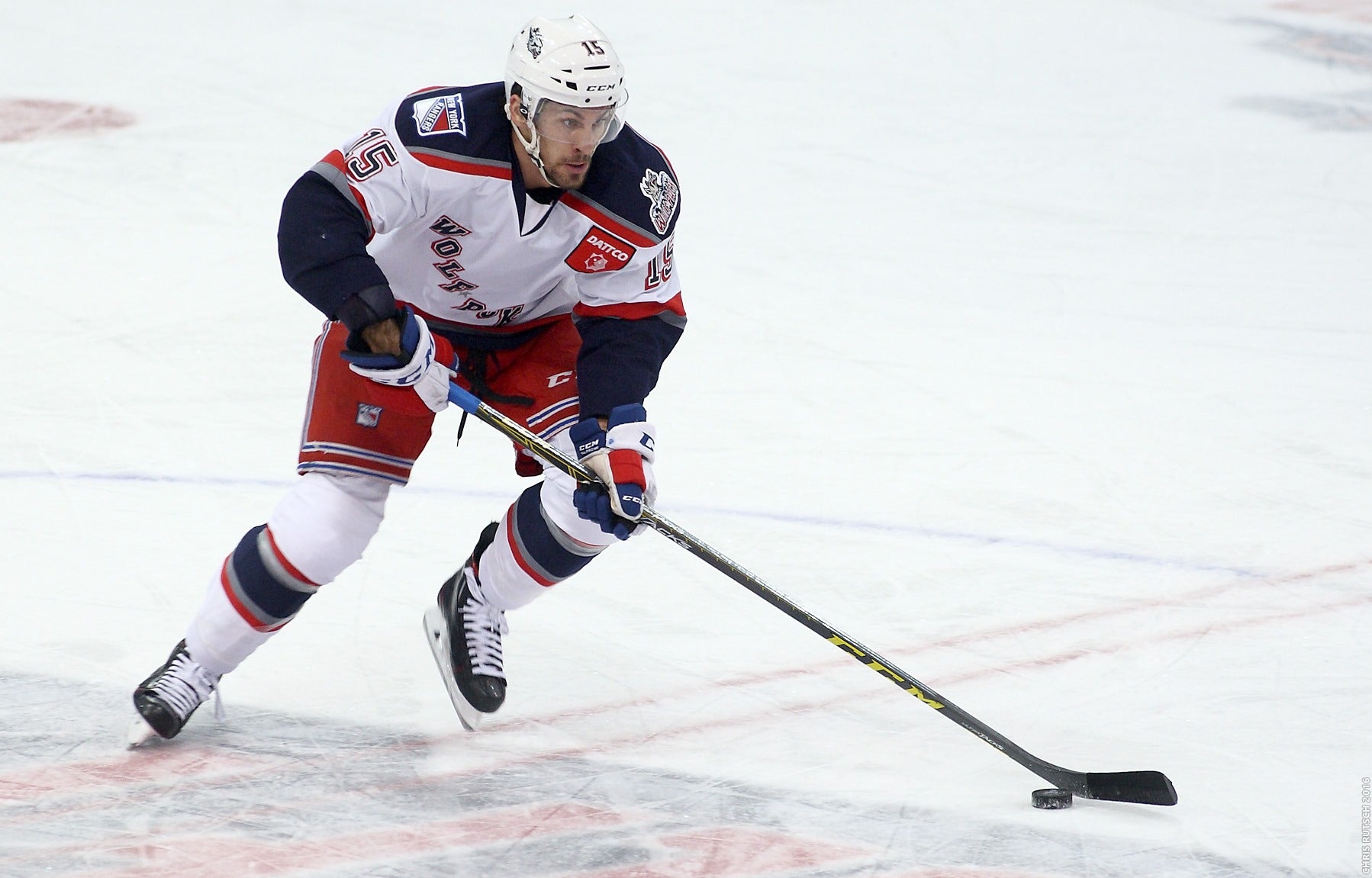This photograph captures an intense moment on an ice hockey rink, featuring a singular hockey player from the Wolfpack team in an offensive stance. The player, wearing a distinctive uniform consisting of red shorts, blue and red striped leggings, and a predominantly white jersey with blue, red, gray, and black accents, is skating rapidly from left to right. Their white helmet, marked with the number 15 and a wolf head logo, includes the text "C&M" on the front, adding a touch of personalization and distinction. The player's aggressive lean and the forward reach of their long hockey stick are evidence of their control over the puck, which is visible on the bottom right of the image, suggesting a swift, decisive movement. Notably, they seem to be alone on the ice, indicating that this could be a practice session or a penalty shot scenario. The inclusion of a New York Rangers patch on the shoulder hints at an affiliation with the major league team, reinforcing the player's professional training and skill level.